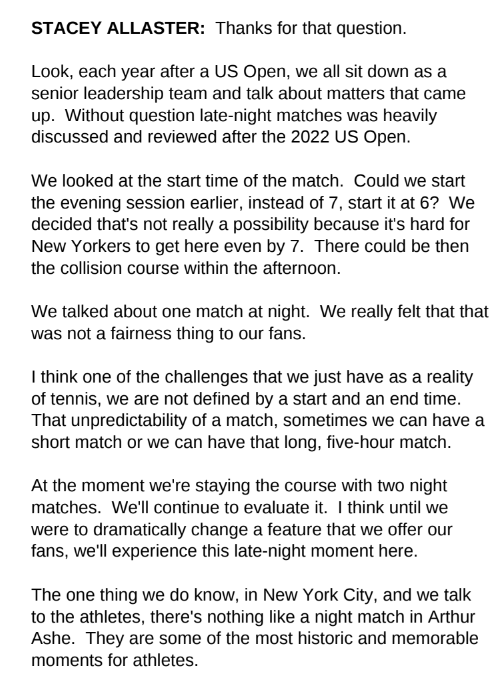This image is a black-and-white text document in portrait orientation with left-aligned text. The document features the heading "Stacy Allister" in bold text followed by "thanks for that question." in medium weight text. There are six paragraphs forming a narrative about the US Open. The text, written informally as if in conversation, addresses the aftermath of the 2022 US Open. It elaborates on discussions by the senior leadership team, specifically regarding the logistics of night matches. They considered starting the evening sessions earlier but concluded it was impractical due to the difficulty for New Yorkers to arrive by 7 PM, let alone 6 PM. The team also reviewed the fairness of having only one night match but maintained the importance of offering two night matches despite the unpredictability of the game’s duration—from short matches to lengthy five-hour contests. The document emphasizes the unique and memorable experience of night matches at Arthur Ashe Stadium, highlighting their historic significance for athletes and fans alike.